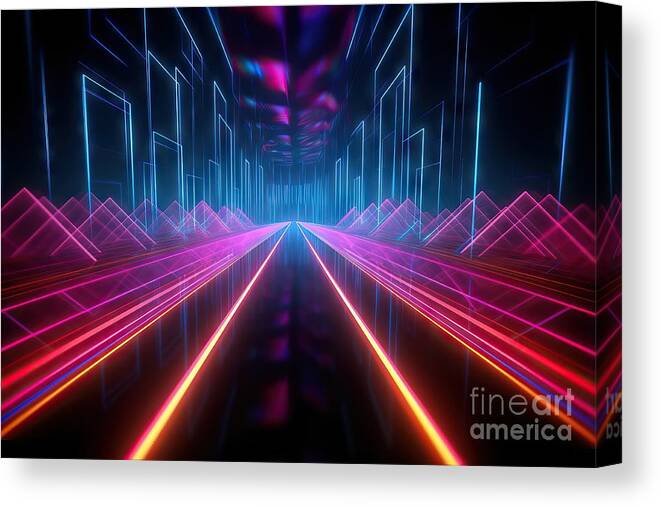This captivating piece of digital art, imprinted with "Fine Art America" in the bottom right corner, presents a mesmerizing array of geometric and colorful lights against a completely black background. The image resembles a long, symmetrical hallway or pathway formed by two parallel lines of bright orange-red lights. Flanking these luminous lines are stacks of lights that seem to form semi-transparent barriers reaching about waist height. The artwork features a variety of glowing geometric shapes, including intricate arrangements of purple triangles or pyramids. The scene appears to extend infinitely, creating an illusion of depth with rows upon rows of varied lights in red, orange, blue, yellow, pink, and purple hues. The ceiling is illuminated by a soft, cloud-like blend of pink, blue, and purple lights, further enhancing the otherworldly atmosphere. This vibrant and meticulously designed composition evokes the feel of walking down a dazzling hallway of multi-colored laser lights, making it an entrancing visual journey showcasing sophisticated modern art.